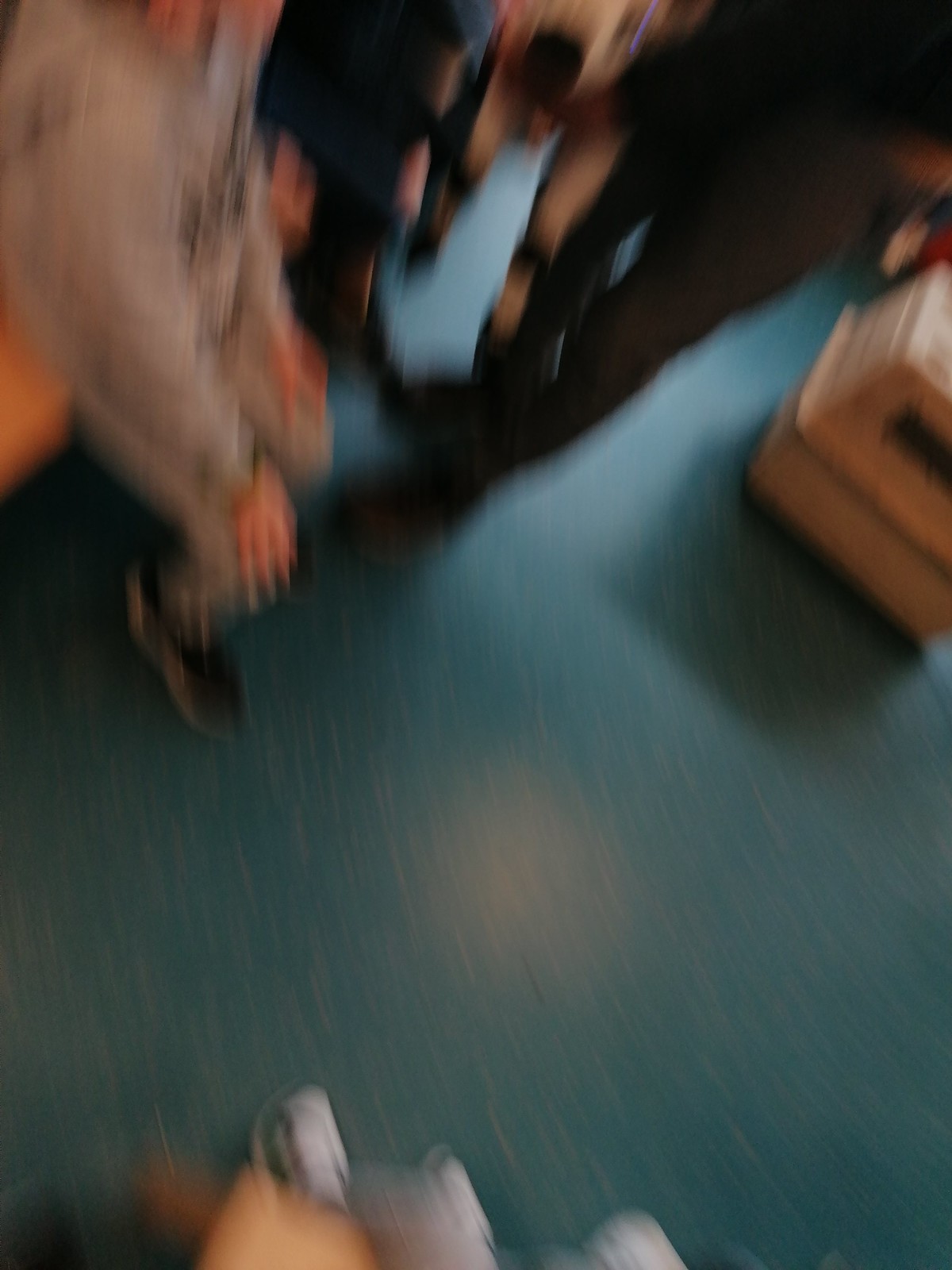The vertically rectangular image is highly blurred, likely due to camera movement during the shot, giving it a dynamic, almost abstract quality. The background, a teal-hued surface, appears to be a floor. At the bottom of the frame, the feet of a person are visible, anchoring the scene. To the right, partially extending into the frame, is a beige animal carrier, hinting at the presence of a pet or transport scenario. In the upper left quadrant, from the shoulders down, a person is seated with their hands resting on their knees, their body oriented towards the right side of the image. The indistinct, motion-filled capture hints at a moment in transition or activity.